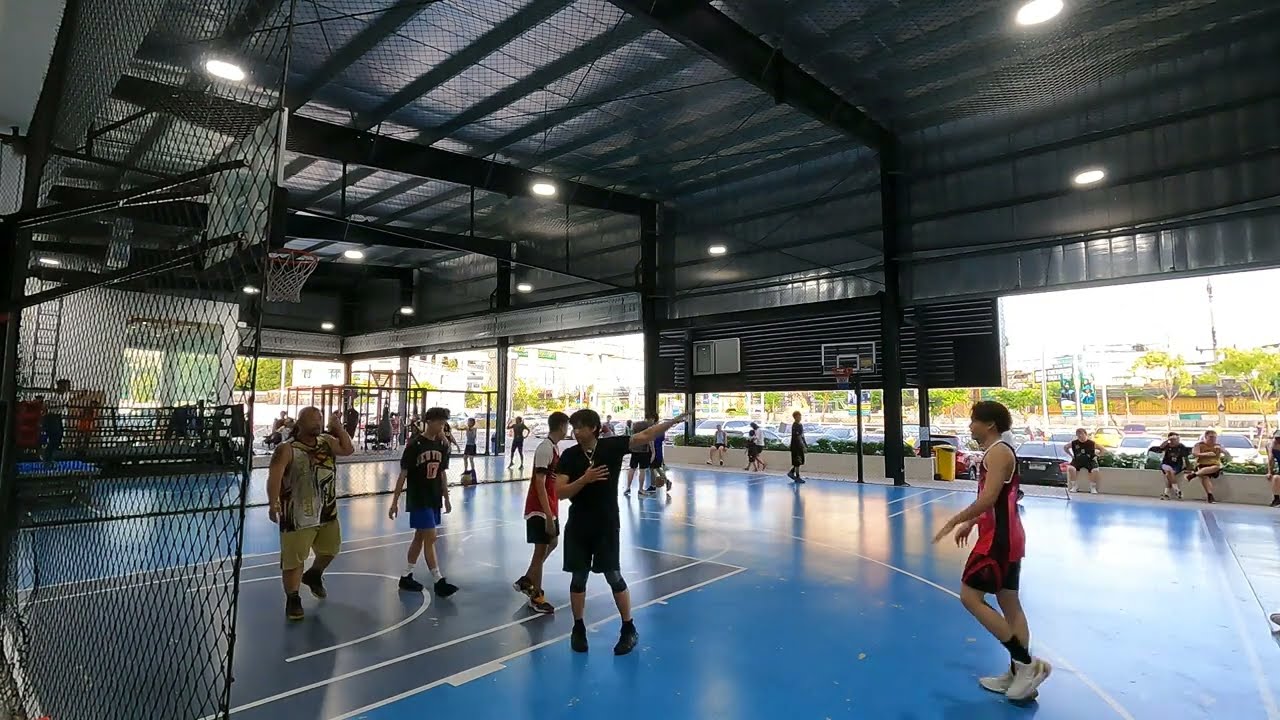In an open-air gymnasium with a blue and black basketball court featuring clear backboards and black hoops, several young men are engaged in intense pickup basketball games. The gym, lacking traditional walls and instead opening out into a parking lot with visible cars and trees, provides a unique recreational space complete with sliding shutters for closure. On the left side of the image, a heavyset man in yellow shorts and black shoes watches near one of the baskets. At the far end, another man is casually shooting hoops alone. In the foreground, a man in a red top with red and black shorts is actively involved in one of the games. Amidst the action, a man who appears to be refereeing has his hand raised, directing the play. A number of people can also be seen sitting and observing the game from the background. This lively scene is possibly taking place in a youth center or a facility like a YMCA, where various sports including boxing are available.